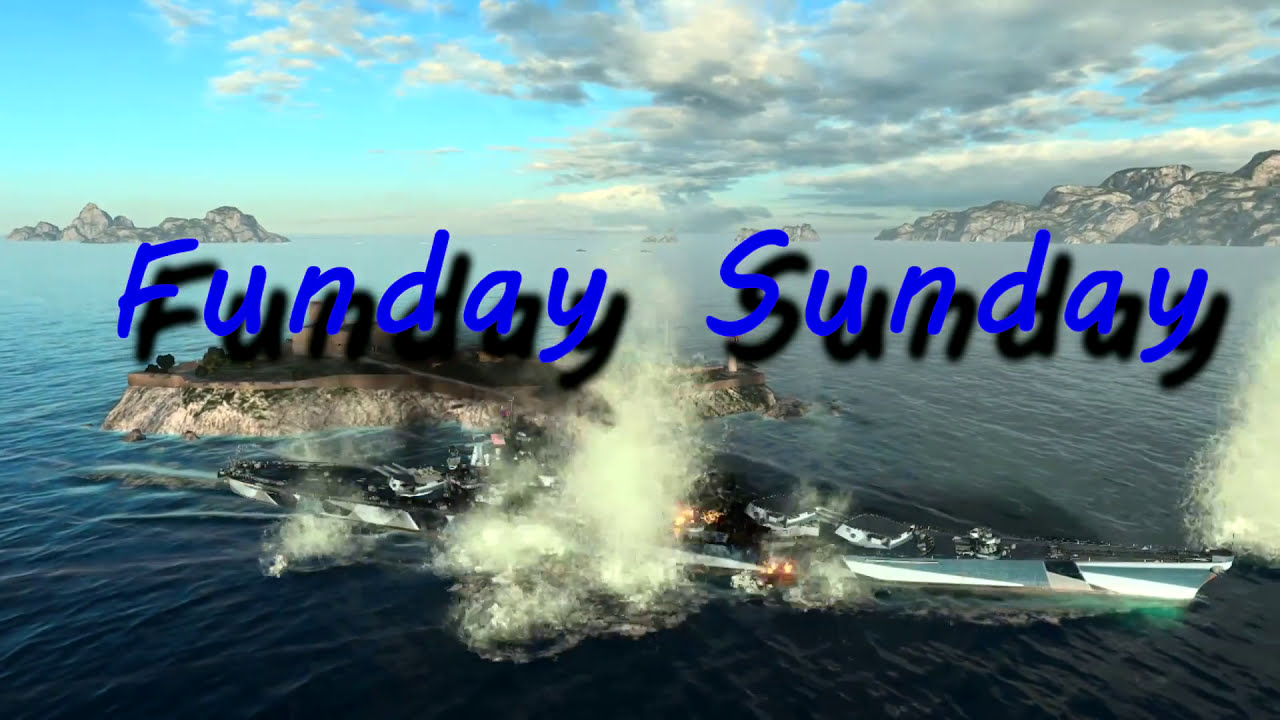The image appears to be an advertisement, possibly for a tropical adventure or a video game, featuring a dramatic maritime scene. The backdrop showcases a sparkling, azure ocean on a partly cloudy day, with scattered, stone-filled islands adorned with lush green vegetation. The sky on the left is clear, giving way to gradually denser cloud formations as you move right. A striking feature is a small island in the foreground, with a high plateau or cliff jutting out of the water. 

Prominently in the center of the image, a large speedboat or battleship is seen, adorned with aqua blue and white stripes, and bristling with impressive gun turrets. The boat is surrounded by water explosions, adding a dynamic and thrilling element to the scene. Above this action, in bold blue Comic Sans font with a black shadow effect, the text "Fun Day Sunday" stretches across the image, emphasizing a promotional or leisure activity theme.

In summary, the image skillfully combines elements of a serene tropical setting and high-octane nautical action, making it an appealing advertisement for an adventurous "Fun Day Sunday."